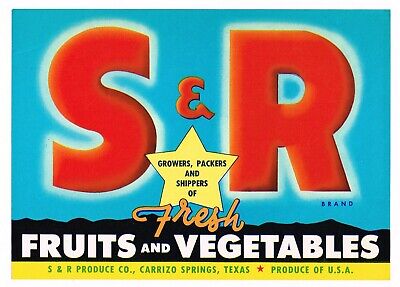This vibrant advertisement features the S&R Produce Co from Carrizo Springs, Texas, known for being growers, packers, and shippers of fresh fruits and vegetables. Dominating the center of the image, large bold red "S&R" letters with white borders prominently display "brand" underneath in nearly tiny black text. Above this, a yellow-filled star contains the text "Growers, Packers, Shippers of," while the word "Fresh" is elegantly scripted below the star. Further down, "Fruits and Vegetables" is presented in plain white block text, set against a contrasting black background that highlights its clarity. The background of the entire ad is a vivid blue, which emphasizes the bright and engaging design. At the bottom of the image, there is a yellow banner that stretches across with the text "S&R Produce Co, Carrizo Springs, Texas." Adjacent to this is a small red star accompanied by the phrase "Produce of USA," ensuring the viewer knows the origin of the products.